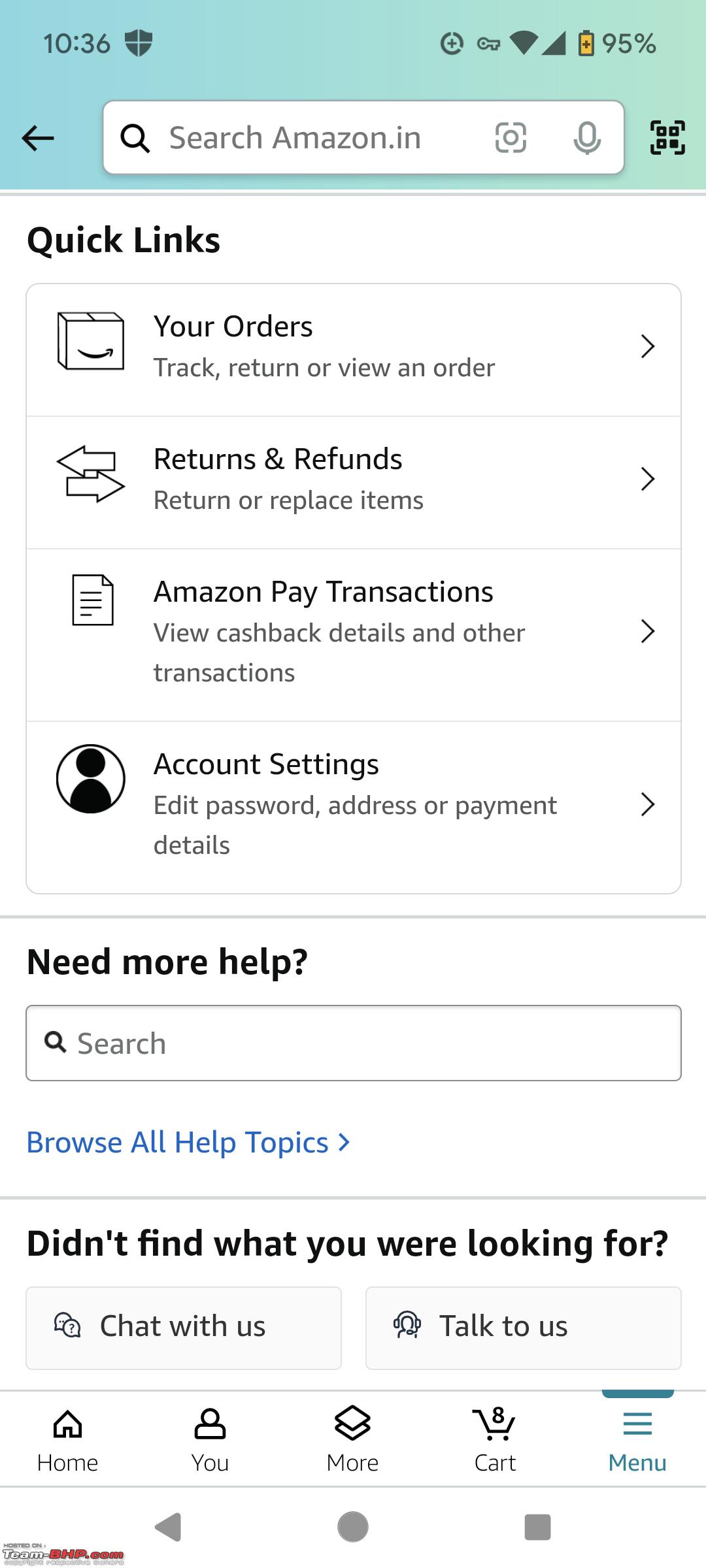The image depicts a mobile phone screen focused on an app interface, displaying various account and help options. At the top, there's a blue status bar showing the time (10:36) and a battery indicator at 95%. Below it, there's a black left arrow icon, followed by a search box and an icon resembling an 'X' within a box.

The main background is white, featuring a section titled "Quick Links" with options organized vertically. The options and their respective descriptions are:

1. "Your Orders" - Track, return, or view an order (with an arrow pointing right).
2. "Returns & Refunds" - Return or replace items (with an arrow pointing right).
3. "Amazon Pay Transactions" - View cashback details and other transactions (with an arrow pointing right).
4. "Account Settings" - Edit password, address, or payment details (with an arrow pointing right).

This section is outlined with a blue border. Beneath it, there is a thin blue line followed by a section titled "Need more help?" which is also outlined in blue. It contains another search box labeled "Browse all help topics" (with an arrow pointing right).

Further down, a thinner blue line separates another prompt asking "Didn't find what you were looking for?" accompanied by two light blue buttons: "Chat with us" and "Talk to us."

At the bottom of the screen, a navigation bar is present with options: Home, You, More, Cart, and Menu, all highlighted in blue. Additionally, there are icons for Back (left arrow), Recent Apps (square), and Home (circle) at the bottom of the interface, accompanied by small gray and red text.